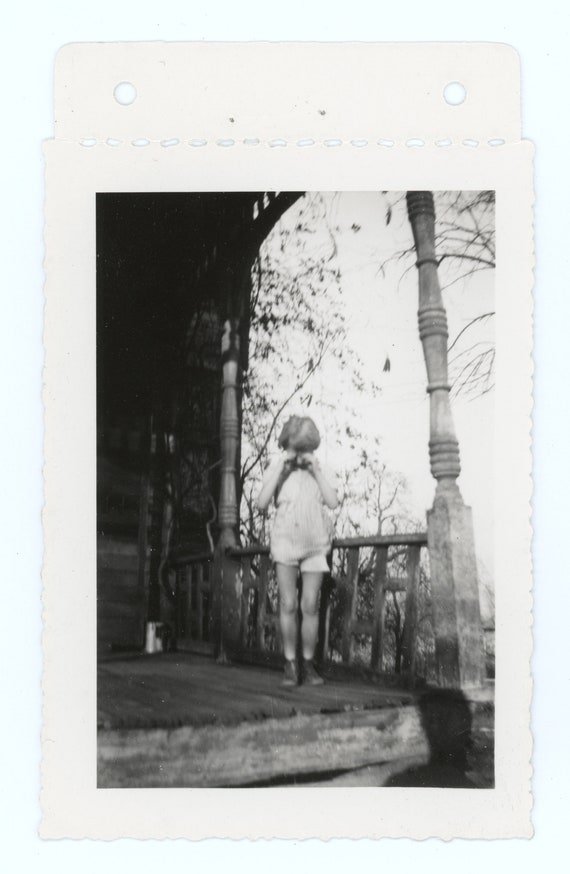This black-and-white photograph captures a distressed child standing on a worn-out wooden porch. The child, whose gender is indeterminate, is dressed in a white linen outfit consisting of short sleeves, shorts, and shoes. The child is visibly upset, with hands balled into fists and pressed against tear-filled eyes, appearing to rub away the tears. Behind the child, there's an ornate railing that seems to have been turned on a lathe, adding a touch of craftsmanship to the otherwise dilapidated setting. The wooden porch shows signs of wear and tear, indicative of age, with the backdrop featuring some trees and the shadow of the person taking the photograph. The entire image has a soft, hazy quality, suggesting that it could either be an authentic old photograph or a digitally altered one to appear vintage. Overall, the scene evokes a somber, melancholic mood.